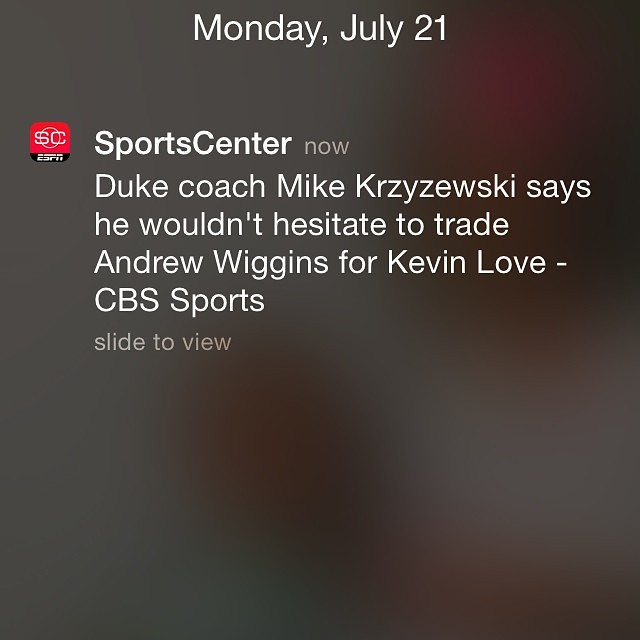The image is a square screenshot from a mobile phone displaying a tweet-like notification from Sports Center, posted on Monday, July 21st. The background is primarily dark gray with spots of red towards the top and center, adding a hint of color along with the Sports Center logo. At the top in white text, it reads "Monday, July 21." Below that, a small red square logo with rounded edges features the letters "SC" in white, encircled in the center, and accompanied by the ESPN logo in white on a black background. Next to the logo, it says "Sports Center" followed by "NOW" in light gray. The main content of the notification, in white text, reads: "Duke coach Mike Krzyzewski says he wouldn't hesitate to trade Andrew Wiggins for Kevin Love - CBS Sports." Beneath this, in light gray, it says "Slide to View," indicating that swiping would reveal more content. The overall look is simple yet informative, typical of mobile notifications.